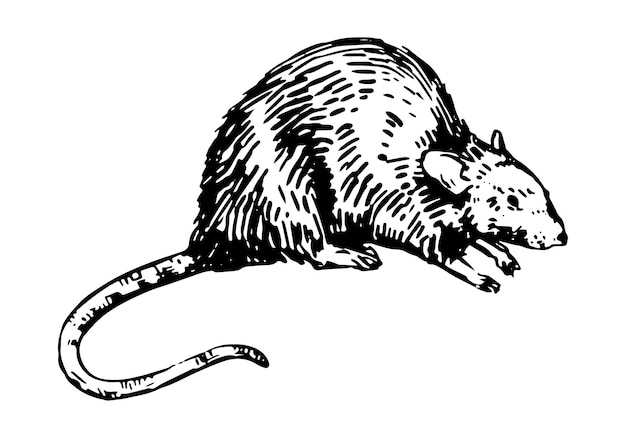This image is a monochrome illustration of a rodent, possibly a mouse or a rat, depicted in black and white. The image primarily features the rodent's side profile, facing slightly towards the right. The background is stark white, emphasizing the detailed black shading that defines the rodent's form. The rodent's fur appears sleek, and its long tail, ears, and single visible eye are all meticulously rendered. There is intricate detailing on the feet, showcasing tiny fingers. Despite the absence of text, the illustration is rich in nuances, such as the black dot on the nose and the closed mouth. Notably, the image does not include whiskers, and the rodent appears alone with no additional elements in the composition.